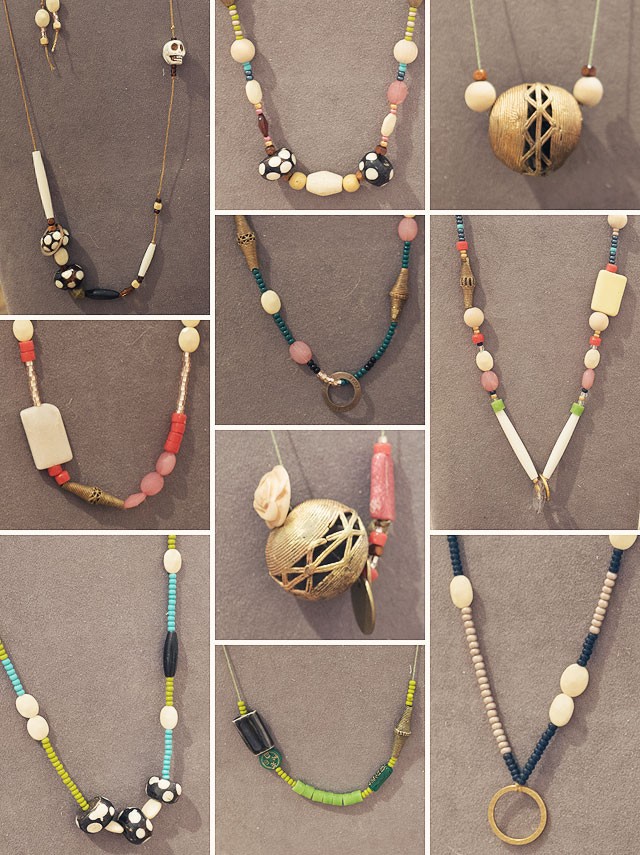The vibrant image showcases a vertically rectangular collage made up of 10 individual photographs, each separated by a white border. Each photograph displays a unique, beaded necklace, arranged neatly in three vertical columns – three on the left, four in the middle, and three on the right.

Starting from the left column, the necklaces include one with long white beads, another featuring a skull on a gold chain, and a third combining white and coral beads. The middle column begins with a piece adorned with a mix of white, pink, and dotted black beads, followed by one with turquoise seed beads and larger white and pink beads. A large gold sphere necklace is positioned above a simpler one made up of chartreuse and lime green beads.

In the right column, a large gold sphere necklace stands out, flanked by large wooden or cream-colored beads. Below this, a multicolored necklace and another with cream and navy hues complete the collection.

The necklaces vary widely in design, featuring an array of beads and stones in colors like dark blue, light green, lime green, yellow, light blue, black, pink, red, brown, tan, beige, and dark teal. The photo, taken straight on, captures the necklaces either laid flat or hanging, giving a clear view of their intricate details and design variety.